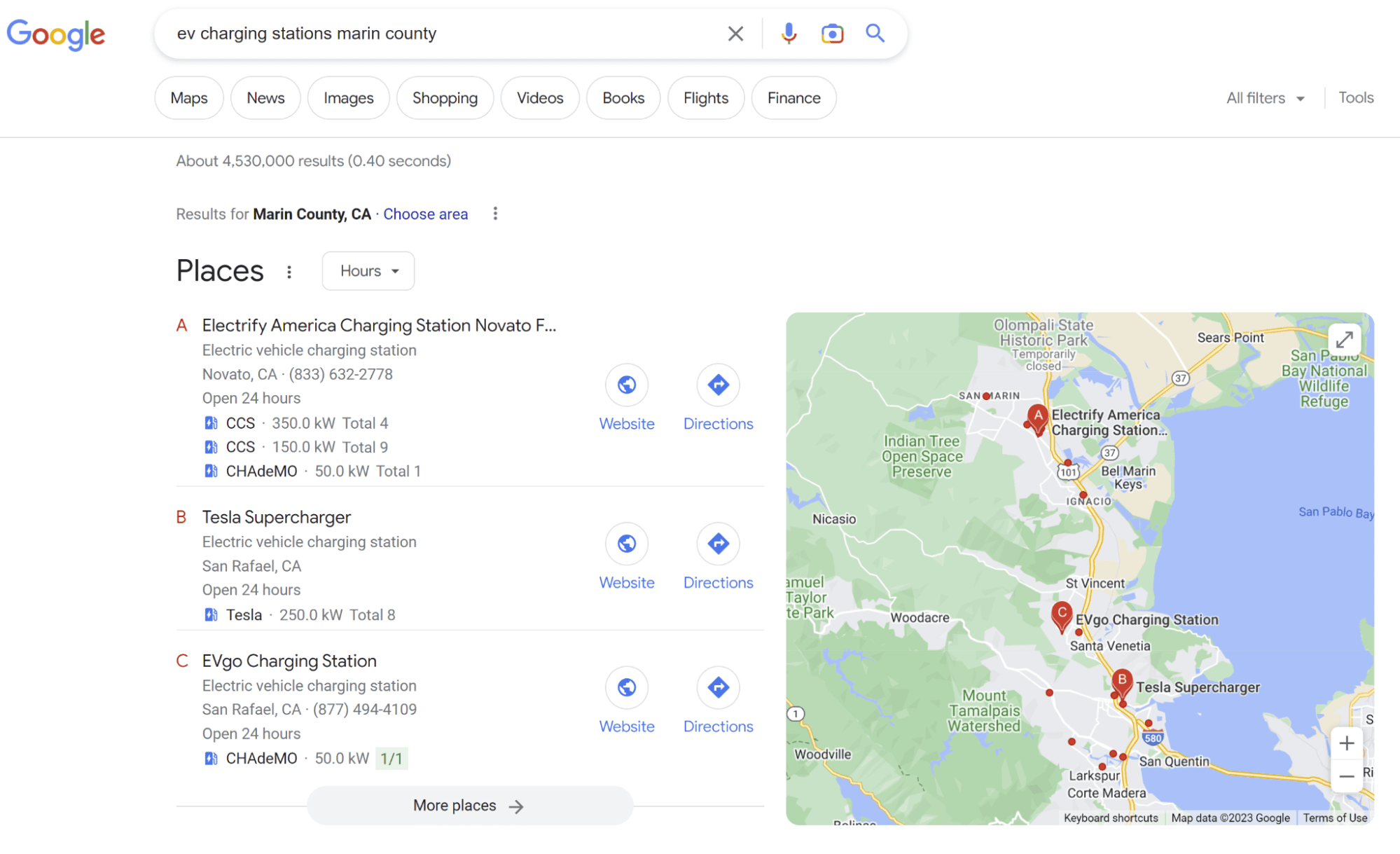A detailed caption for the described image could be:

"The image showcases a Google search results page for 'EV charging stations' in Marin County. At the top-left corner, the Google logo is prominently displayed in its signature blue, red, yellow, and green colors. Below the logo, the search bar contains the query 'EV charging stations Marin County,' accompanied by an 'X' for clearing the search, a microphone icon for voice search, a camera icon for image search, and a magnifying glass icon to perform the search. Directly beneath the search bar are navigation buttons labeled Maps, News, Images, Shopping, Videos, Books, Flights, and Finance.

Towards the right, there is an 'All Filters' dropdown menu and a 'Tools' button separated by a thin line. The search results display 'About 4,530,000 results (0.4 seconds)' immediately below these options. The next section highlights 'Results for Marin County, California, CA,' with a clickable, blue-highlighted 'Choose Area' prompt. Adjacent to this is a small map with red pins indicating specific locations, mostly centered around a water body. 

Following the map, there are listings labeled A, B, and C, each providing location details for the identified EV charging stations."